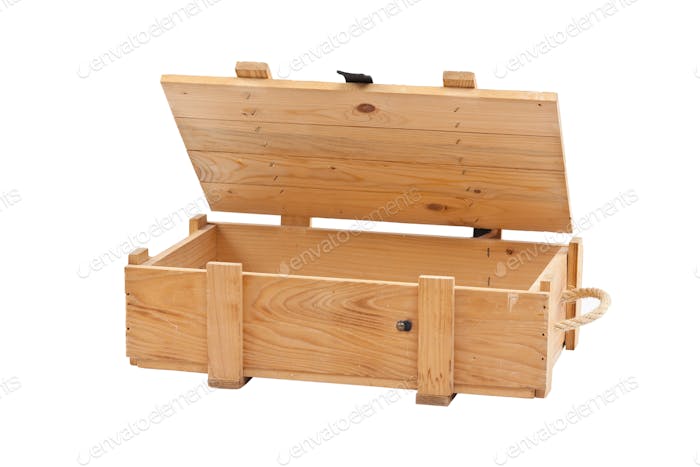The image depicts a rectangular wooden box made from light-colored wood, possibly pine, showcasing the natural gradients of the wood grain. The box is constructed from wooden planks and reinforced with vertical wooden supports. It features rope handles made of beige or cream-colored rope on the sides, designed for easy dragging. The lid of the box is partially open and is attached with a hinge and a clasp, although the clasp's exact connection point is unclear. The box's construction includes nails or staples visible at the underside where slats are attached to the top, sides, and bottom, indicating sturdiness. The entire image is watermarked with "Envato Elements," appearing in multiple rows and partially obscured due to its light lettering.